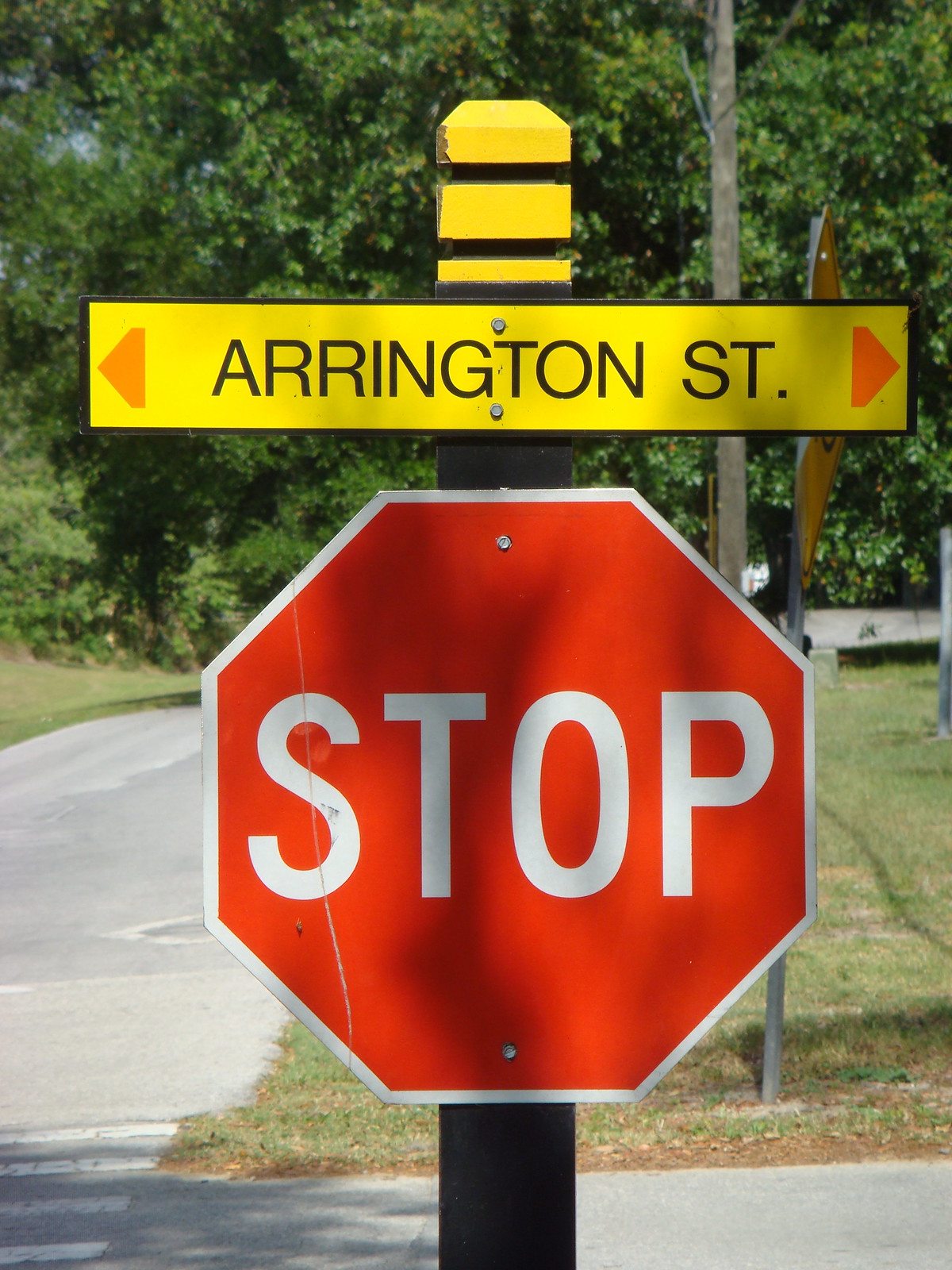The image depicts an American stop sign, prominently positioned on a black metal pole. The red, octagonal stop sign features a white border and the word "STOP" in bold white letters. The sign is securely fastened to the pole with visible silver rivets. Affixed above the stop sign is a yellow rectangular sign that reads "Arlington Street" in black letters, accompanied by two orange arrows indicating directions left and right. The upper part of the black pole is painted yellow in sections for high visibility. The photograph appears to be taken from a close distance, about three to four feet away. In the backdrop, tall trees are visible lining the road, alongside a driveway curving to the right, suggesting a residential area. Another sign, possibly a stop or yield sign, can be seen behind the main structure.